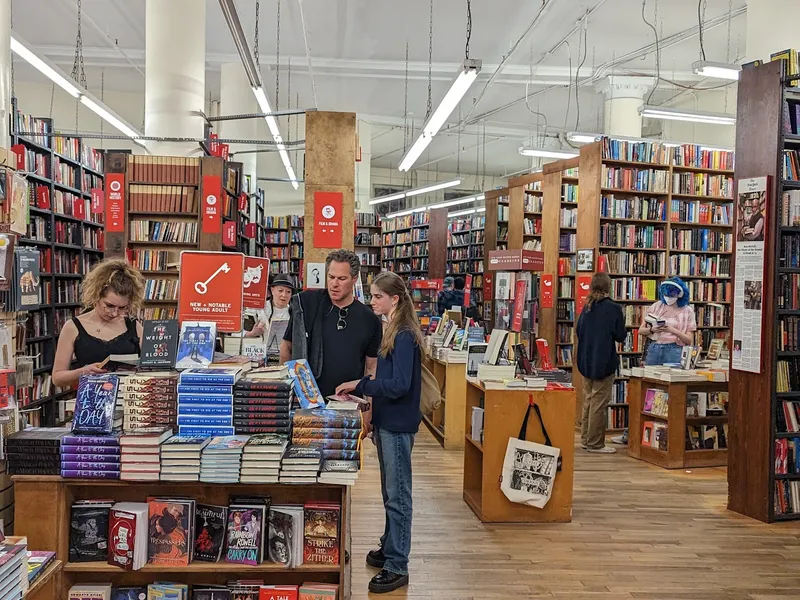The image captures the interior of a cozy bookstore bustling with activity. A minimum of seven people can be seen throughout the space. Most of the visitors appear to be women, with one man in a black shirt and sunglasses also present. Surrounding them are numerous shelves filled to the brim with books of all genres, neatly organized. A wooden floor adds warmth to the setting. Positioned to the side is a small stand with a tote bag hanging from it. The bookstore features white pillars supporting the ceiling, which is adorned with large rectangular fluorescent lights, casting a bright and inviting ambiance. Red signs with catchy designs, including one with a key motif, add pops of color and guide readers through the store.